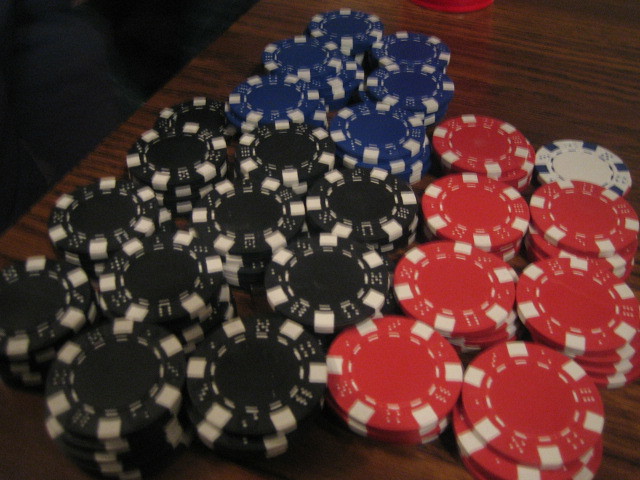This is a color photograph of a large assortment of casino-style poker chips arranged on a dark brown wooden table, possibly made of cherry or mahogany, with visible wood grain. In the top left of the image, there are six stacks of blue chips, each featuring a blue center and alternating blue and white edges. On the bottom left, there is a significant pile of black chips, organized into eleven high stacks, notably taller than the blue ones. The lower right of the image features three rows of black chips, while just above this section, there are two rows of red chips, with a total of seven stacks. Towards the top right corner, there is a solitary white chip standing out from the rest. The table's rich reddish-brown hue provides a striking contrast to the vibrant colors of the poker chips, enhancing the image's overall depth and detail.